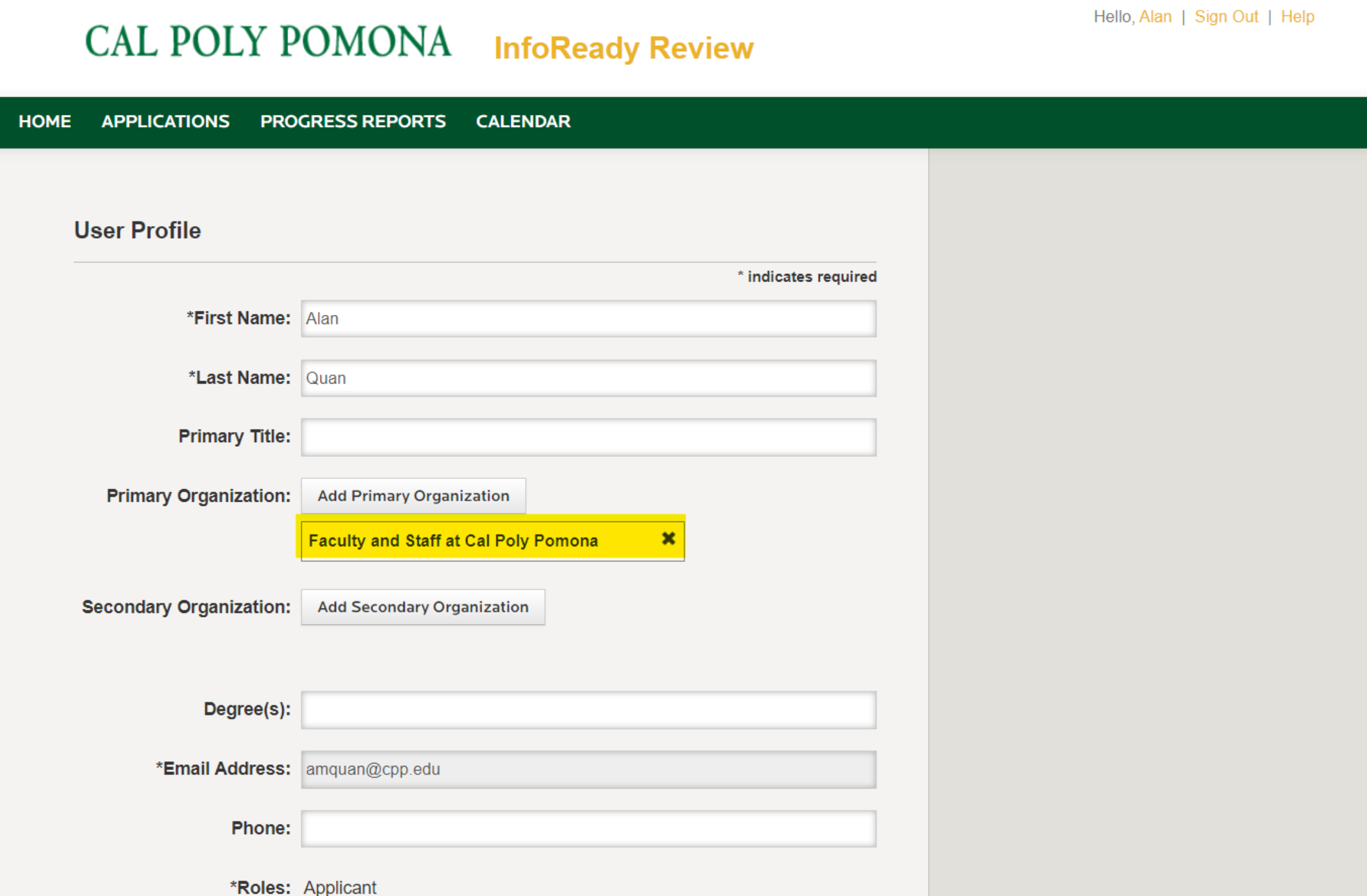Screenshot of an online application form for creating a user profile within the database interface of Cal Poly Pomona. The interface features a title with dark green text reading "Cal Poly Pomona," adjacent to "InfoReady Review" in orange text. The top-right corner displays a greeting that reads, "Hello, Alan," along with options for signing out and accessing help. Below this, a green navigation bar provides quick links to "Home," "Applications," "Progress Reports," and "Calendar."

The main content area, set against a light gray background with a darker gray border, prominently displays a section titled "User Profile." This section includes multiple fields such as "First Name," with the entry "Alan," and "Last Name," with the entry "Kwan." Additionally, fields for "Primary Title," "Primary Organization," "Secondary Organization," "Degrees," "Email Address," "Phone," and "Roles" are also visible. A button labeled "Indicates Required" signifies mandatory fields within the form.